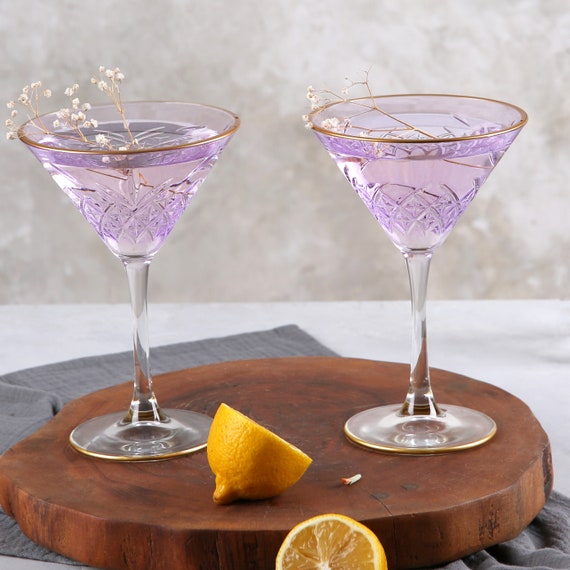In the image, there are two elegant martini glasses filled with a light lilac or purple drink, each adorned with a delicate sprig of baby's breath. The glasses, featuring ornate designs and gold rims, are placed on a rustic, circular wooden platter that showcases the natural grain and dark brown stain of the wood, complete with visible rings and branch nubs. Accompanying the drinks are two lemon halves, one on the platter and the other next to it, cut side facing towards the viewer. This wooden platter rests on a dark grey cloth, which in turn is set on a pristine white marble table. The background is a blurry shade of grey or beige, enhancing the focus on the beautifully arranged drinks and their accompanying elements.